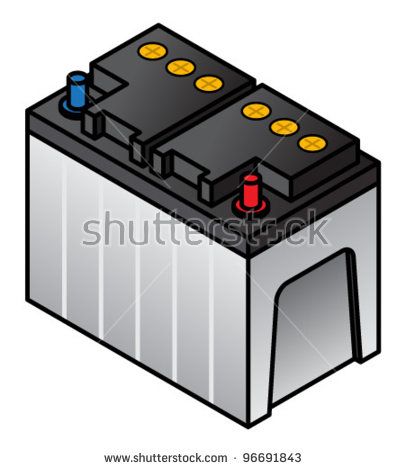The image depicts a stock photo of a car battery against a solid white background, identifiable by the grey "Shutterstock" watermark across its center and the website URL at the bottom that reads "www.shutterstock.com 966-91843". The battery is rectangular in shape with a light gray base and black edges. The front of the battery features thin vertical white stripes adding to its design. The top section of the battery is solid black, and it includes two sets of three yellow circles, each marked with plus signs – one set on the left and the other on the right. At the upper left corner of the battery's top is a protruding blue knob, while a similar red knob is situated at the upper right corner. The meticulous detailing and structured appearance of the battery components enhance its functional aesthetics.